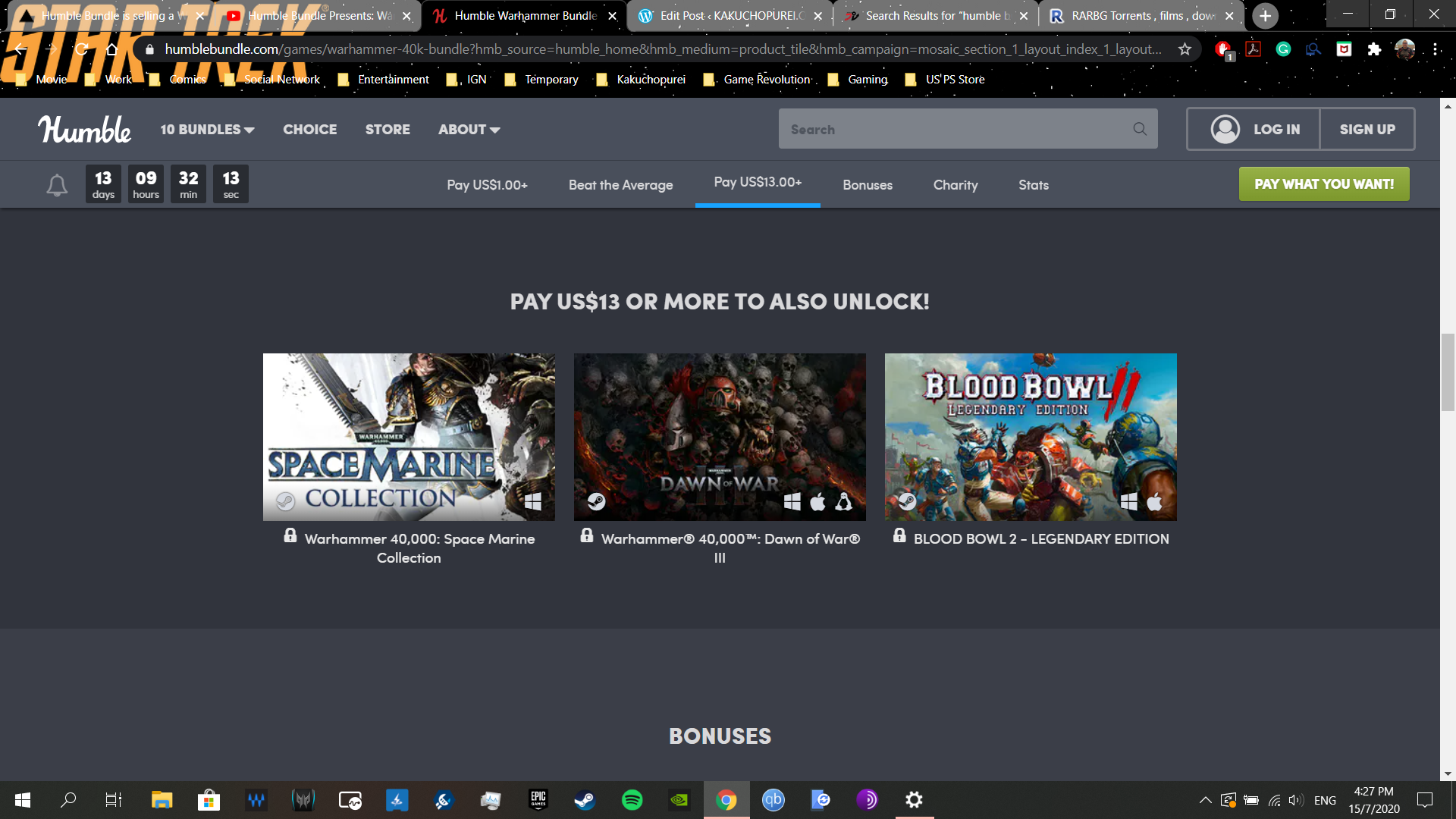This is a screenshot of a laptop displaying an online store website specializing in the sale of various games. The website features a dark background with prominent white text, creating a clear and visually striking contrast. Several game titles are showcased, including "Space Marine," "Dawn of War," and "Blood Bowl." The website offers a unique purchasing model where users can choose to pay what they want to access and play these games, either by downloading them or unlocking them for online play.